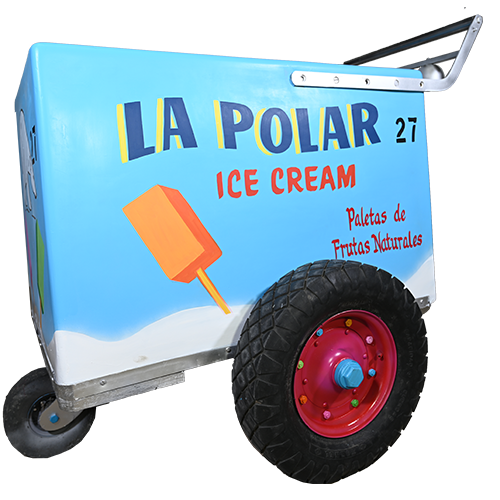The image depicts a rectangular, metal, light blue ice cream cart typically pushed around in urban areas for distributing ice cream. It features a distinct white curvy section at the bottom resembling a cloud and a large black tire at the back with a burgundy red rim, light blue bolt in the center, and colorful screws in pink, orange, and green around the rim. The cart's front sports a smaller black rubber caster wheel attached to a black metal bracket. Painted prominently on the side is an orange, rectangular popsicle with a yellow stick. Above the popsicle, in blue letters with a yellow drop shadow, it reads "La Polar" and next to it, in black text, is the number "27." Below this, the words "Ice Cream" are written in red, and further down, to the right, the phrase "Paletas de Frutas Naturales" appears in red text. A large silver handle is bolted to the side, curving behind the cart for easy pushing. The entire setup rests against a simple white background.